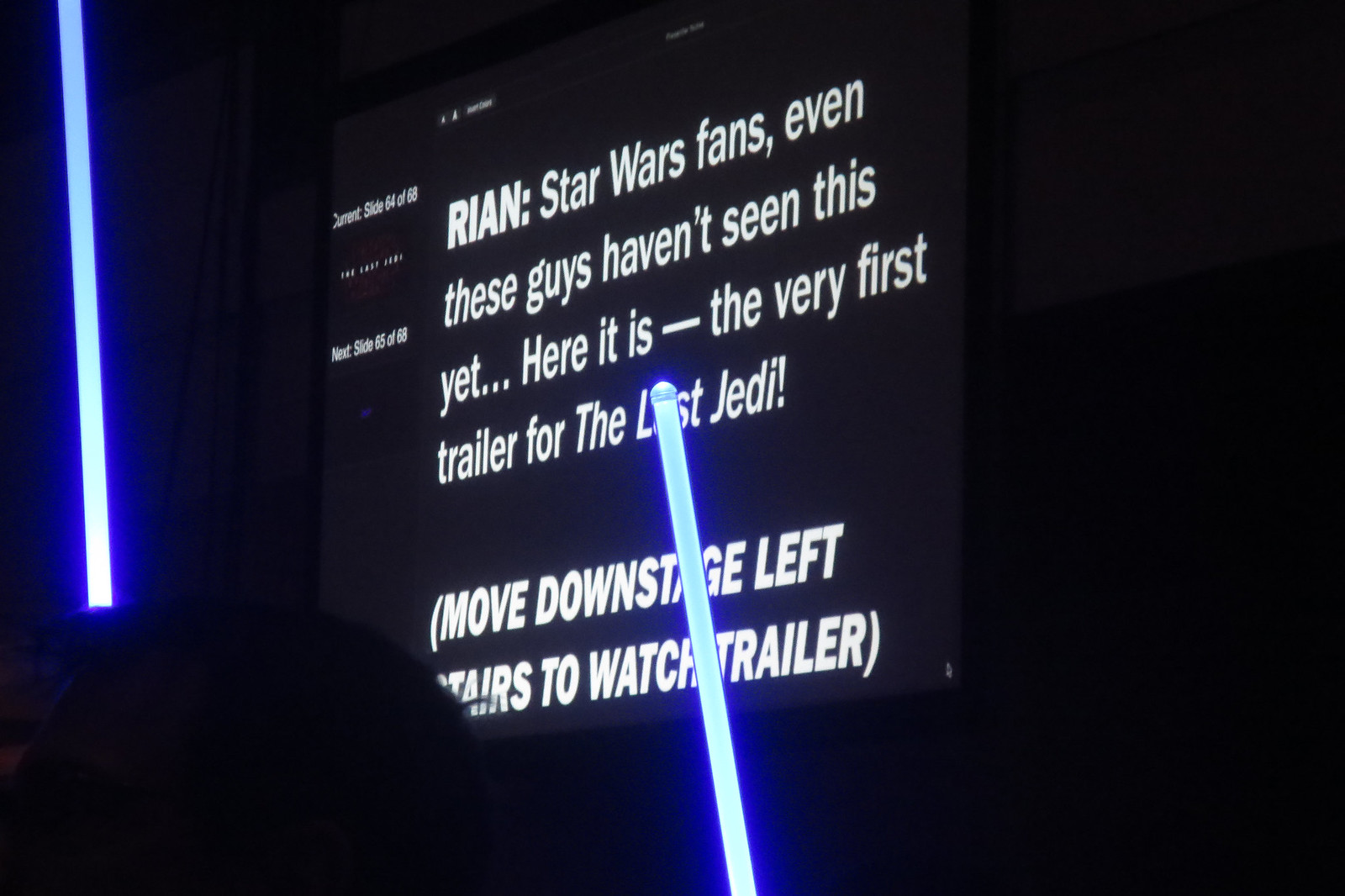This detailed color photograph, captured in landscape orientation, portrays a dimly lit scene with a screen displaying white text against a subtly distinguishable black background. The setting appears to be a movie theater or studio, characterized by the profound darkness that envelops the environment. In the foreground, two neon-blue, tubular lightsabers extend from the left side and the center of the image, brilliantly illuminating their immediate surroundings.

The screen text reads: "Rian: Star Wars fans, even these guys haven't seen this yet... Here it is - the very first trailer for The Last Jedi!" Below this, an additional line in all caps within parentheses states: "(MOVE DOWNSTAGE LEFT STAIRS TO WATCH TRAILER)." Noticeably, there is a dark object, possibly someone's head, partially obscuring the bottom left corner of the image. Additionally, the edges of the screen are faintly visible, slightly lighter than the encompassing black. On the side of the screen, a slide sequence is indicated: "Current slide, 64 of 68, The Last Jedi. Next, slide 65 of 68," hinting at the progression of a presentation.